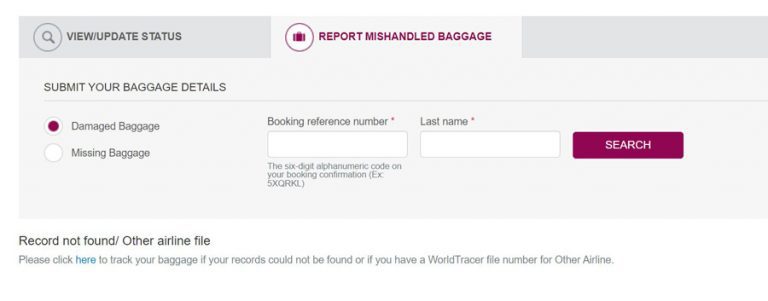A screenshot of an airline's online portal for reporting mishandled baggage is displayed on a computer monitor. The website prominently features an interface where users can report lost or damaged luggage. The page's key elements include sections to submit details such as the booking reference number, which is typically a six-digit alphanumeric code found on the booking confirmation, and the passenger's last name. The page uses a color scheme of gray and maroon, with instructions highlighted in maroon, including the option circled to indicate 'damaged baggage'. 

At the bottom, a maroon-colored search bar allows users to proceed with their report. If the initial search yields "Record not found", users are provided with an additional link to track baggage through other airline files using a World Tracker file number. The comprehensive layout of the portal aims to simplify the reporting process for passengers dealing with mishandled baggage.